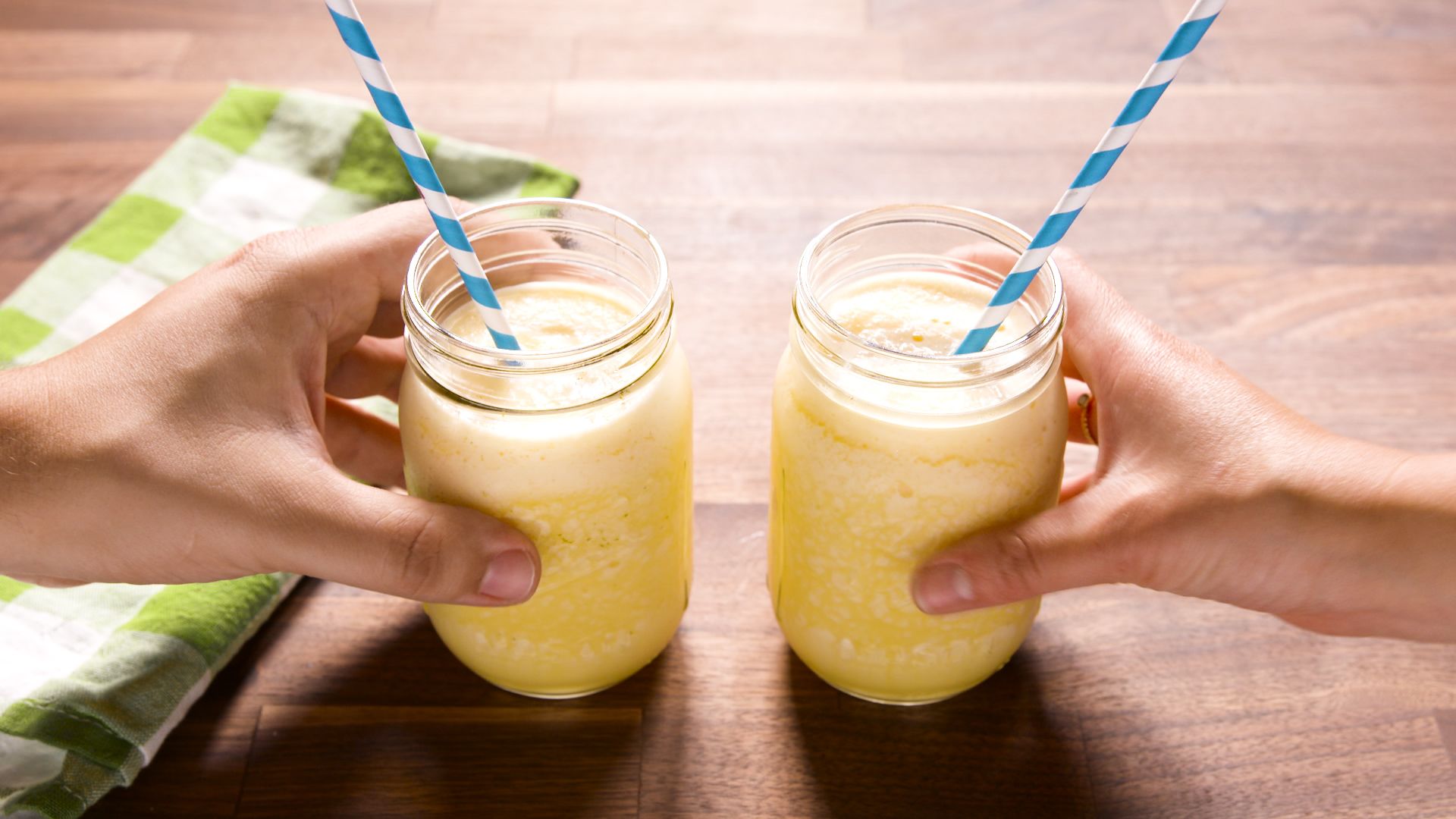The image depicts two mason jar glasses, each filled with a thick, pale yellow liquid topped with a creamy white froth, suggestive of a milkshake or smoothie. The mason jars, sitting almost evenly spaced apart on a wooden table with visible slats, are held by a pair of Caucasian hands—one jar in a smaller right hand and the other in a slightly larger left hand, each grasped between the thumb and index finger. Both jars feature light blue and white ribbed paper straws. To the left side of the mason jars, a checkered dish towel, with alternating squares of green and white, lies folded on the table, adding a touch of rustic charm to the setting.